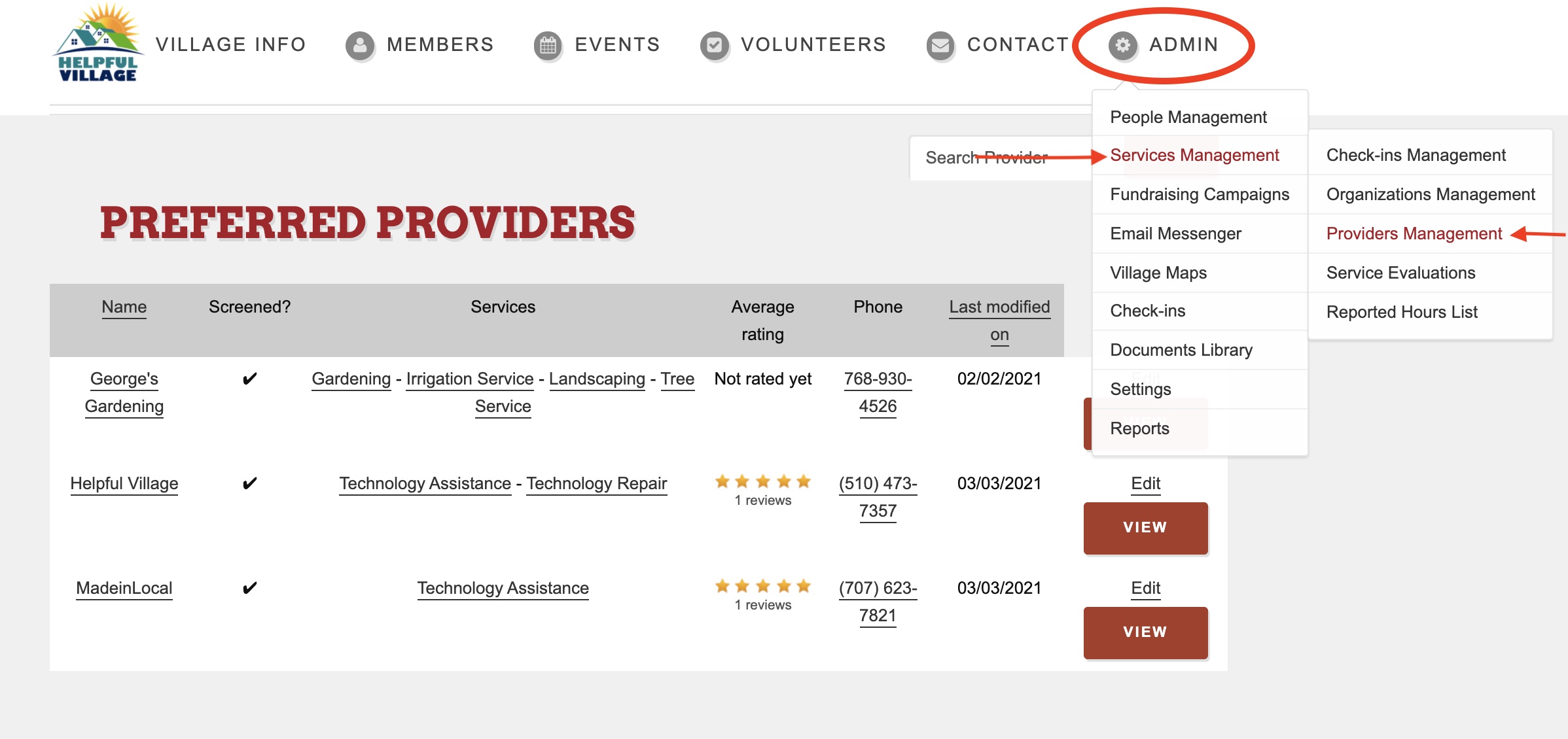This image depicts the admin interface of a community management platform called "Helpful Village." The header of the portal lists several navigation tabs, including "Village Info," "Members," "Events," "Volunteers," "Contact," and "Admin." The interface appears to be designed for administrative use, as indicated by a red-circled "Admin" label at the top. 

The central portion of the image displays a list of service providers identified under "Preferred Providers," including "George Gardening," "Helpful Village," and "Made in Local." Each provider entry includes details such as services offered, ratings, phone numbers, and the date of the last modification.

Additionally, the image features a dropdown menu, likely serving as a tutorial or guide. This menu is organized into two sections: the main dropdown and a mini dropdown. The main dropdown encompasses options such as "People Management Services," "Fundraising," "Email Messages," "Village Maps," "Check-ins," "Documents Library," "Settings," and "Reports." The mini dropdown further decomposes into "Check-ins Management," "Organizations Management," "Providers Management," "Service Evaluations," and "Reported Hours List."

The color scheme of the admin portal is predominantly white with an off-shell white background, creating a clean and organized interface. This detailed view exemplifies a robust setup for managing community services, payments, and various maintenance tasks.